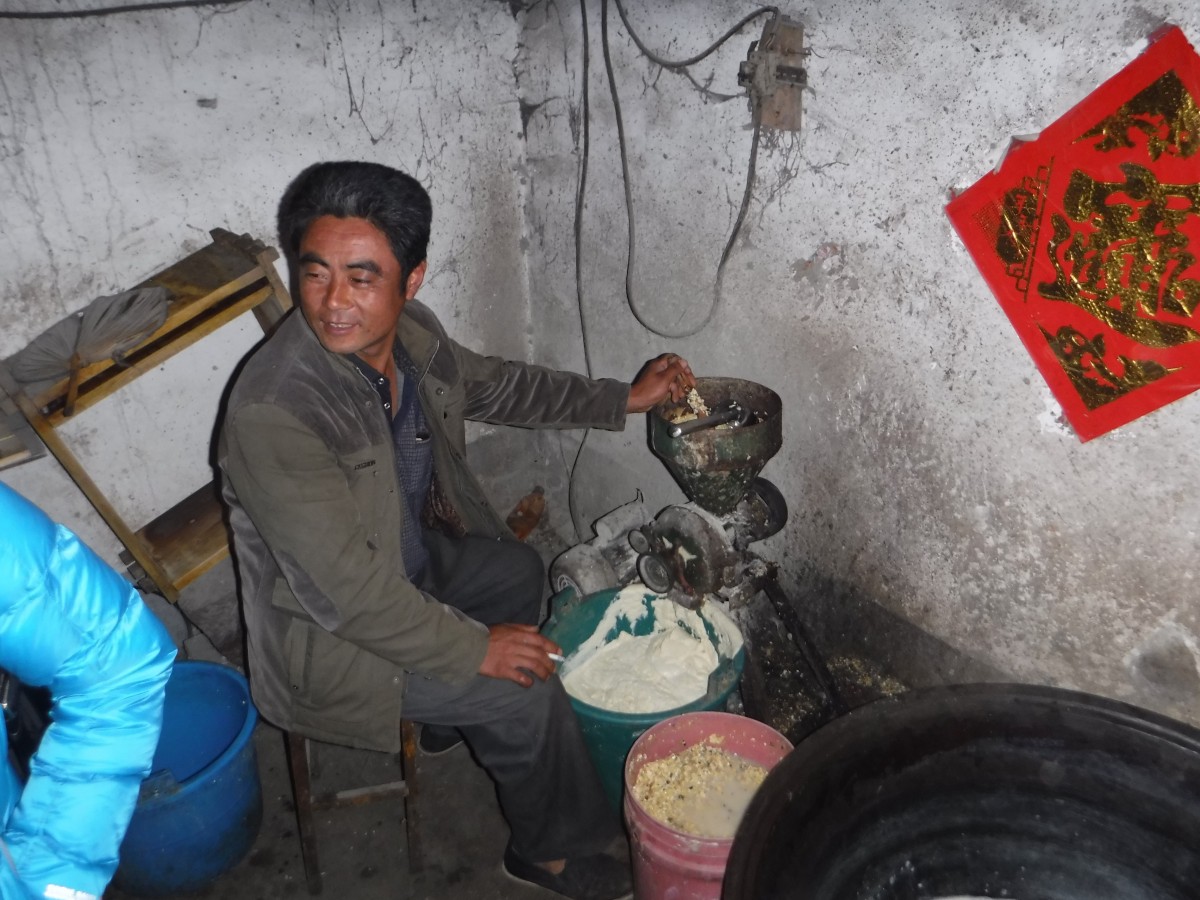In this detailed color photograph, taken indoors in a dilapidated, basement-like room, an Asian man is sitting on a wooden stool in the corner, engaging with a contraption that appears to be a grinder, likely for processing corn or a similar grain. The walls are made of concrete and covered in cobwebs, contributing to the gritty atmosphere. The man, who seems to be in his mid-30s, is smiling and looking over his right shoulder, possibly speaking to another person whose arm, clad in a blue parka, is partially visible in the lower left corner. He holds a cigarette between his fingers on his right hand, which rests on his knee, while his left hand operates the grinder. The machine dispenses a white creamy paste or mush into a green bucket positioned beneath it, with a pink bucket containing corn or grain placed nearby. Adding color and cultural context to the scene, the upper right-hand corner of the room features a red diamond-shaped sign adorned with gold, Asian lettering. Adjacent to this is a scarf or banner that might represent a flag or hold religious significance. The man wears an army green jacket, further emphasizing the photo’s raw and authentic feel.